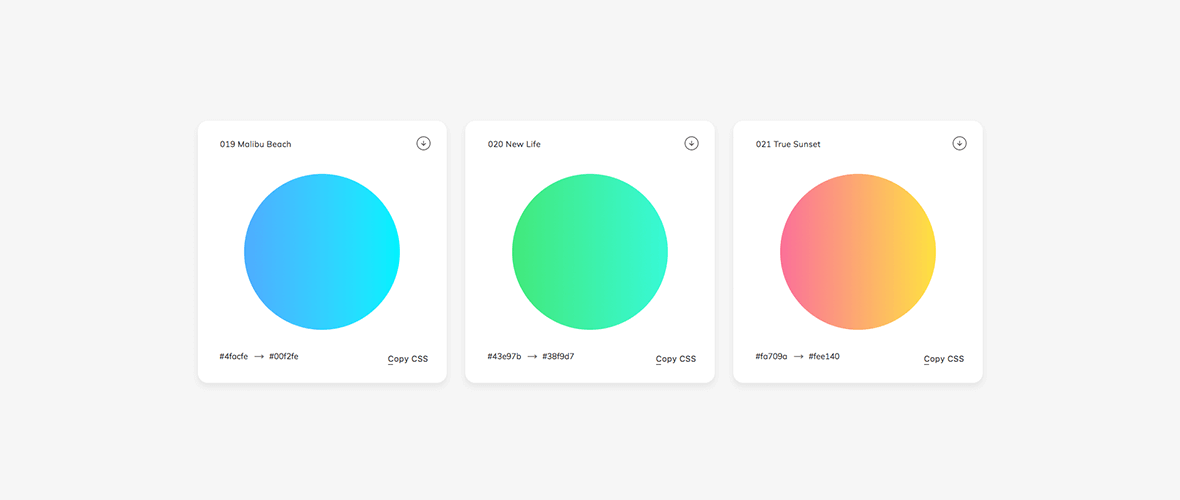The image features a light gray background with three prominent squares arranged in a horizontal row, each with a large circle in the middle. The circle in the leftmost square is light blue, the one in the center square is a teal green, and the circle in the rightmost square has a gradient that transitions from purple on the left to orange on the right. The circles are significantly large, occupying a substantial portion of their respective squares.

In the top left corner of the leftmost square, the text reads "019 Malibu Beach". Within this square, there is a small, indistinct icon enclosed in a circle at the top right corner. Below this, some unclear numbers appear followed by the text "copy CSS". 

The central square has the text "020 New Life" at the top. Similar to the first, it contains a small, hard-to-discern icon in a circle in the upper right corner, with some numbers displayed below the main text that are too blurry to be readable.

The rightmost square features the text "021 True Sunset" at the top. It also includes a small, ambiguous icon encased in a circle at the top right, with additional unreadable numbers below the main text.

Overall, the image is characterized by its geometric simplicity and vibrant color scheme, with each square and circle combination presenting a unique visual and textual element.